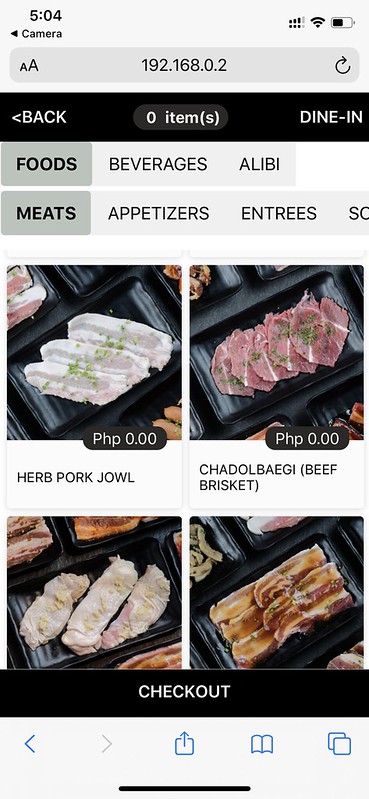This is a highly detailed screenshot of a mobile ordering menu from a restaurant displayed on a smartphone. The top of the screen shows the system status bar: the time is 5:04 AM/PM, displayed in black text on a light gray background that spans the entire width of the phone. On the right side of this bar, three out of four signal bars are visible, indicating network strength, alongside a fully connected Wi-Fi signal, and a horizontal battery icon displaying approximately 50% charge.

Below this, the left side of the screen displays the word "Camera" with a left-pointing triangle arrow, seemingly indicating a previous interface. The next line features a rounded, darker gray rectangular address bar or search bar suggestive of a browser, with a small "A" and a large "A" indicating text size options, an IP address "192.168.0.2" in the center, and a refresh button on the right.

The main UI of the food ordering app begins beneath this, with a black bar running across the top. This bar includes a navigation button labeled "Back" with a left arrow on the left side, "0 items" displayed in white on a dark gray oval in the center, and "DINING IN" in capital white letters on the right.

Following this, the background transitions to white with a top row consisting of three tab-like selections: "Foods" in bold black letters on a dark gray background, "Beverages" in normal black font on a light gray background, and another tab that appears to display "Alibi," also in normal weight letters on a light gray background.

The row below contains more menu categories in a horizontal scroll-like arrangement: "Meats" in bold black text on a dark gray background, "Appetizers" on a light gray background, "Entrees" similarly on a light gray background, and partially visible text starting with "S" and "O," which the image cuts off.

Farther down, the menu displays item images. A PHP (Philippine Peso) 0.00 price tag is shown under an image of what appears to be herb pork jowl in a tray. Next to it are slices of meat in a black tray labeled "PHP 0.00" followed by the title "Chattel Baggy Beef Brisket." Below are two more images of food items, side by side in black trays, one of white meat in three pieces and the other of brown meat, both titles are not visible.

At the very bottom of the screen is a black bar stating "Checkout." The lowest part of the screen displays phone navigation buttons: a left-pointing arrow, a right-pointing arrow, an exit icon, a book icon, and a copy icon.